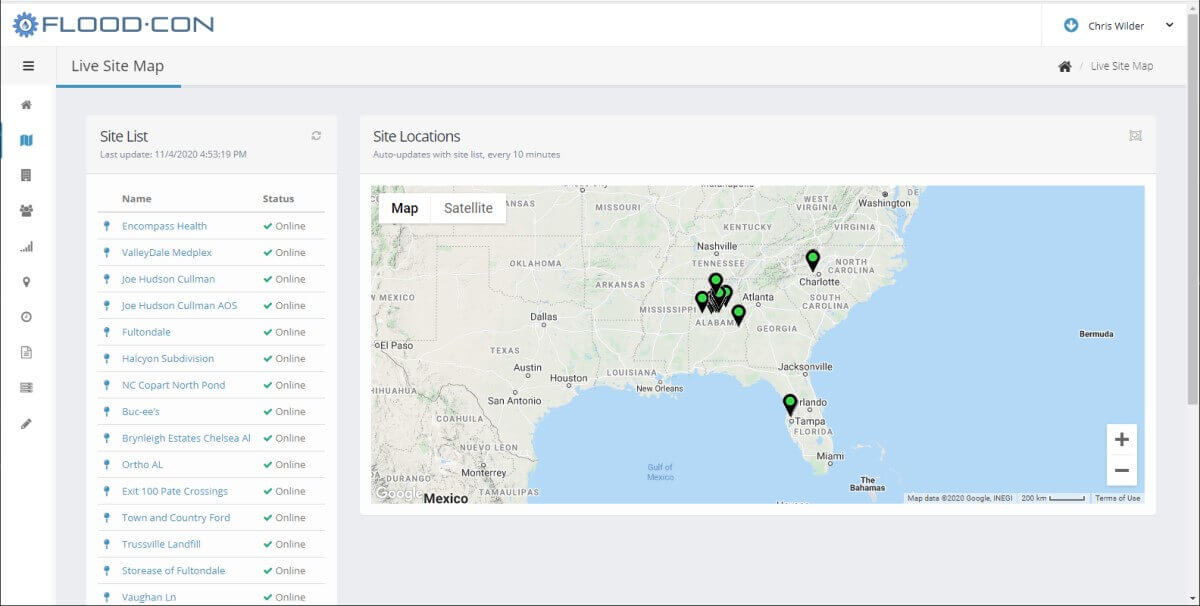At the top-left corner of the webpage, there is a blue emblem resembling a sun, accompanied by the text "flood.com" in blue. Directly beneath, a light gray horizontal rectangle spans the width of the page, displaying the text "Live Site Map." On the right end of this gray bar, there is a small house icon indicating the homepage; beside it, some words that appear too small to read, possibly spelling "side" or "sides."

On the left side of the page, a vertical column is laid out. At the top of this column, there is a gray rectangular section labeled "Site List." Below this, a white rectangular section contains the labels "Name" and "Status." Under this section, a list of names in blue text is visible, each accompanied by a blue checkmark signifying their online status.

To the right side of the webpage, a map is displayed showing various states including Texas, Louisiana, Mississippi, Alabama, Georgia, and Florida, as well as parts of Mexico. The map highlights different cities within these states, marked with pins. At the top of the map, a white rectangular box contains the options "Map" and "Satellite" in black text. In the bottom-right corner of the map, situated over the water, there are plus and minus buttons for zooming in and out. The very bottom corner of the page is shaded gray.